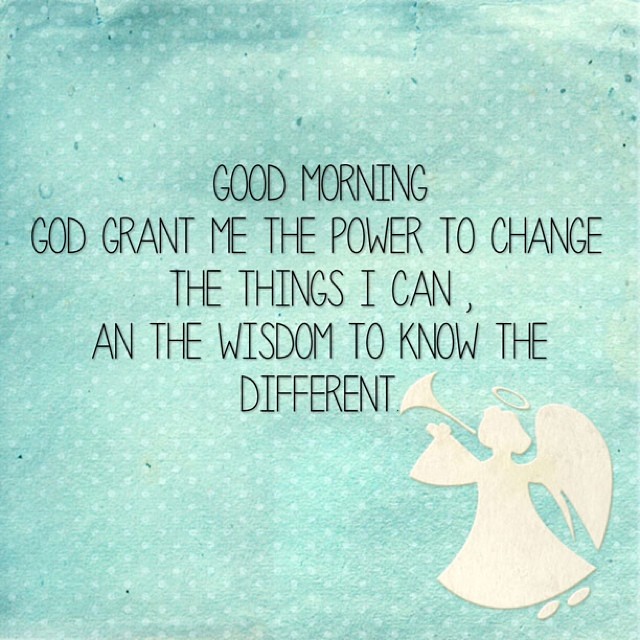The image features a light bluish-green, possibly turquoise, surface adorned with white polka dots. The material appears somewhat worn, reminiscent of aged paper or fabric. In the center, written in black text, is an inspirational message that reads: "Good morning. God grant me the power to change the things I can and the wisdom to know the different." Notably, there are typos in the text, with "an" instead of "and," and "different" instead of "difference." Below the text, in the bottom right corner, is a drawing of an angel dressed in white, blowing a trumpet with a halo above its head.